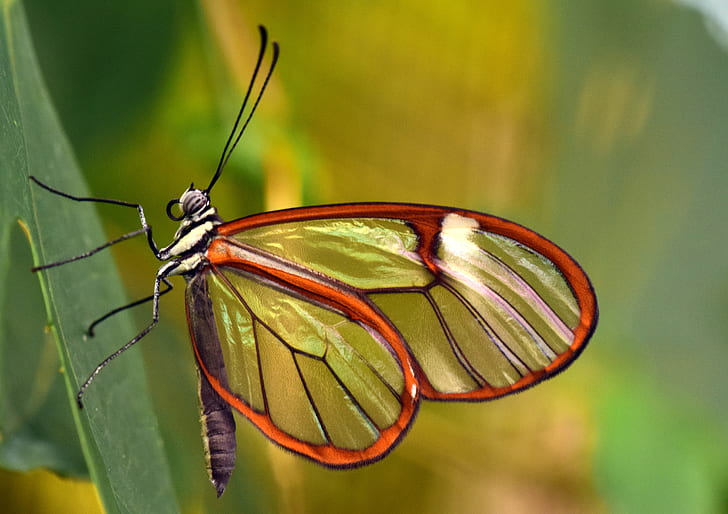This detailed, close-up image captures a butterfly perched on a leaf. The butterfly features transparent wings outlined in orange with intricate black veins running throughout. Its body is notably long, giving the impression of a tail extending from the main body, and it has exceptionally long, black legs and antennae with knob-like ends. The head is small, round, and adorned with two protruding eyes. Although photographed horizontally, the angle suggests the butterfly is climbing, making viewers somewhat cock their heads for a traditional orientation. The background is a blurred mix of green and yellow vegetation, directing full attention to the butterfly's delicate details.